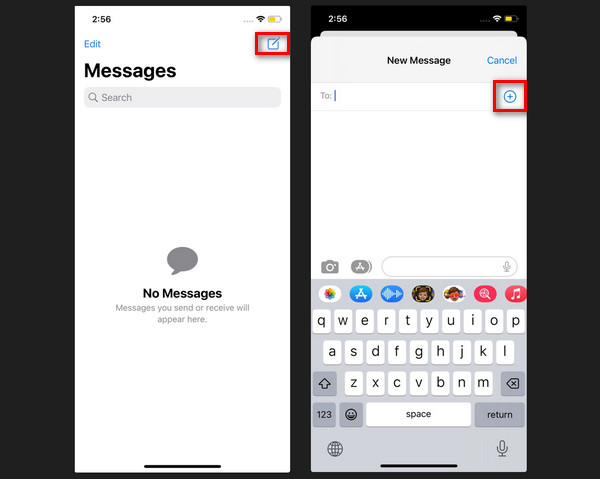A detailed side-by-side comparison of two smartphone user interfaces is displayed. On the left, the screen shows a smartphone layout with a battery indicator at half capacity, fully connected to Wi-Fi, and a 256 label at the top left. The top right features an icon resembling a pen on paper, enclosed within a red user-implemented box. Below this, the screen displays "Messages" heading and a search bar with "Search" in gray text. An empty box follows, stating "No Messages."

On the right, the screen mirrors similar technical details but presents a different interface, likely within the context of a text message. The header is black with "256" in white text. Below, it repeats the "Messages" heading, now combined with a "New Message" label. A "Cancel" option appears to the right in blue, alongside a plus icon intended to add contacts, also enclosed in a red box. Further down, there's a text input bar and a keyboard visible at the bottom. The background of the comparison is a charcoal color, prominently highlighting the two interface screens side by side.